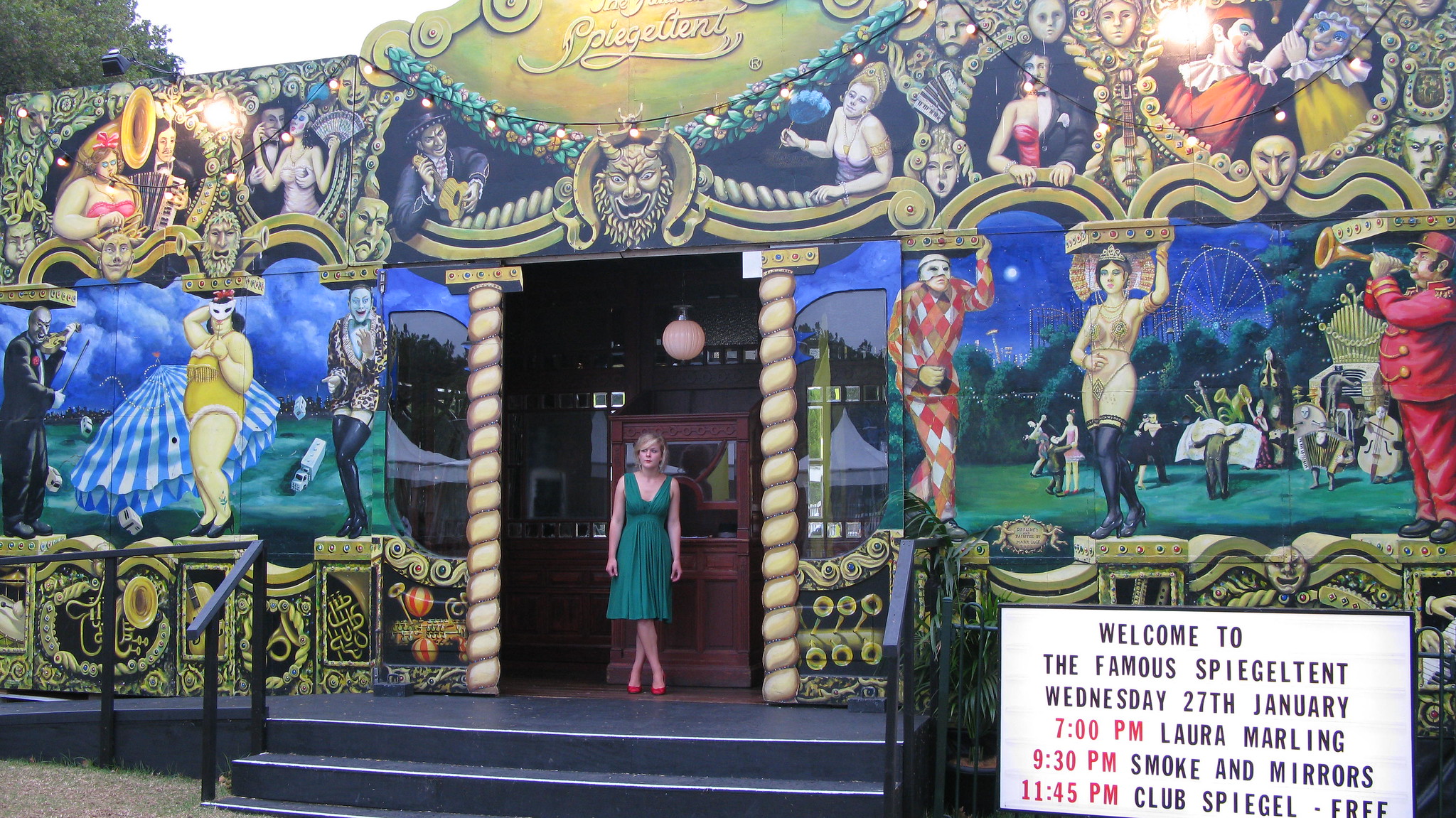In this vibrant and colorful photograph taken outdoors on a sunny day, a blonde-haired woman wearing a V-neck green dress and red shoes is seen standing with her legs crossed, exuding a curious demeanor. She is posed in front of an elaborately painted building entrance that blends the old-world charm of circus sideshows with an ornate mural. The building features an eclectic array of images, including a clown, a woman in a bikini, a man in a red uniform playing a trumpet, and various other intriguing figures. The doorway, accentuated by beveled gold columns, leads up a set of three black stairs and features brown doors. To the right, a prominent white sign painted on the building in black letters details upcoming performances at the famous Spiegel Tent, scheduled for Wednesday, 27th January: Laura Marling at 7 PM, Smoke and Mirrors at 9:30 PM, and Club Spiegel Free at 11:45 PM. The mural’s detailed depictions and the building’s intricate designs create a fascinating backdrop reminiscent of a carnival or circus sideshow, adding a unique, lively atmosphere to the scene.